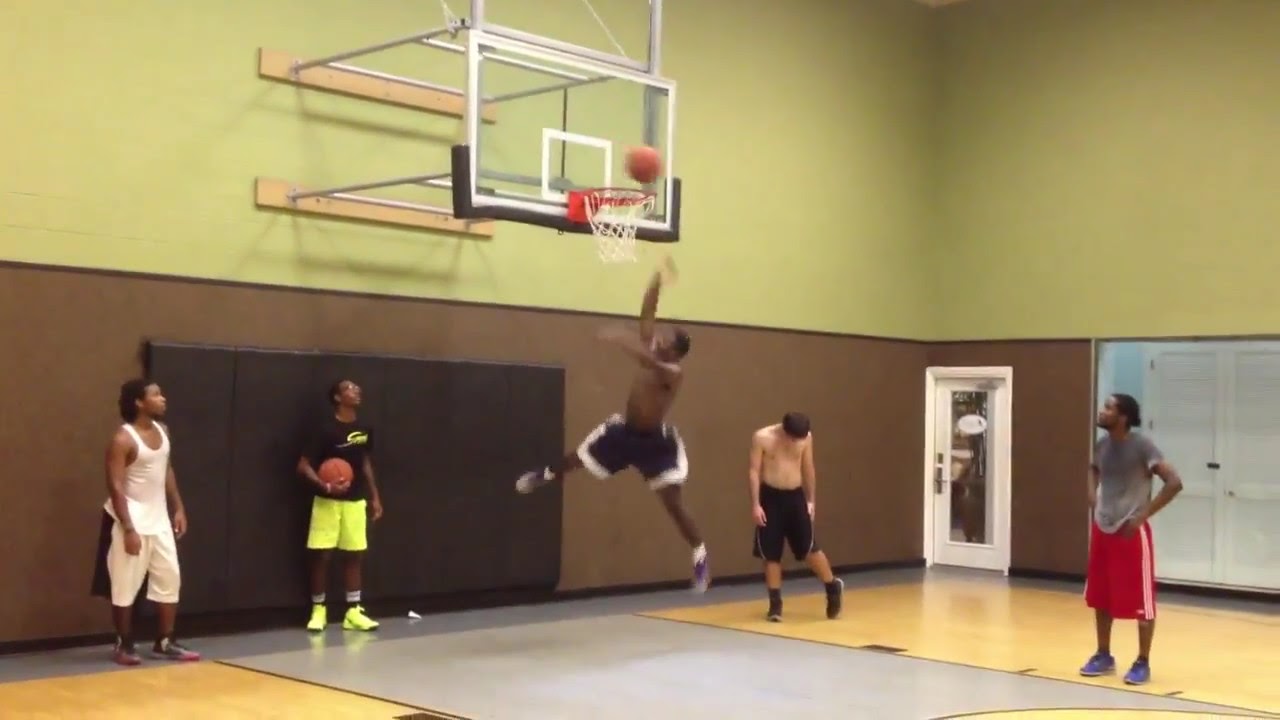In a well-lit, indoor gym with clean, vividly red and yellow-green walls, several young men are immersed in a basketball game on a court with a distinctive gray and yellow-green floor. The image, likely a blurry and pixelated screenshot from a video, centers around a pivotal moment where a young man executes an impressive slam dunk. He jumps remarkably high, his legs splayed wide apart due to the sheer effort of his leap. This player is bare-chested, wearing only black shorts with white trim, and is about to send the ball through the hoop.

Surrounding this dynamic scene are four other players. To his left, a player clad in a black top, lime green shorts, and matching sneakers holds another basketball, while another player in a white tank top and white shorts watches the dunk attentively. To his right, one young man in a gray shirt, red shorts, and blue shoes is also engrossed in the action, while a shirtless player in black shorts and black shoes looks down, distracted from the main event. Of the five players, four appear to be African American, with the fifth being white. The captured moment highlights the athleticism and intensity of the game within this pristine indoor basketball facility.